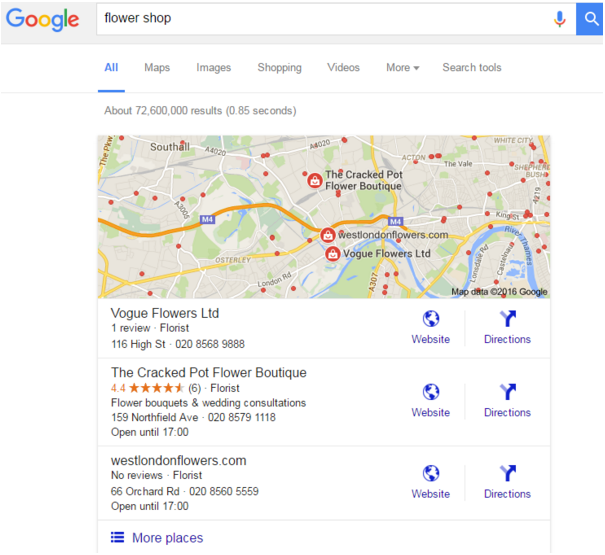The image depicts a Google search results page for the query "flower shop." 

At the top of the page, the iconic Google logo is displayed in its classic multicolor scheme—blue "G," red "O," yellow "O," blue "G," green "L," and red "E." The search bar contains the text "flower shop," with a microphone icon for voice input and a magnifying glass icon signifying the search function.

Below the search bar, there are various filter options: "All," "Maps," "Images," "Shopping," "Videos," "More," and "Search tools," with "All" being currently selected. The page indicates approximately 72,600 search results.

The results feature a map highlighting three flower shop locations and a brief description of each:

1. **Vogue Flowers Ltd.**
   - One review, no star rating displayed.
   - Links to the website and directions.

2. **Cracked Pot Flower Boutique**
   - Rated 4.4 stars based on six reviews.
   - Specializes in flower bouquets and wedding consultations.
   - Open until 17:00.
   - Includes links to the website and directions.

3. **WestLondonFlowers.com**
   - No reviews yet.
   - Open until 17:00.
   - Features links to the website and directions.

At the bottom, users are given the option to click a menu button that expands to show more place options.